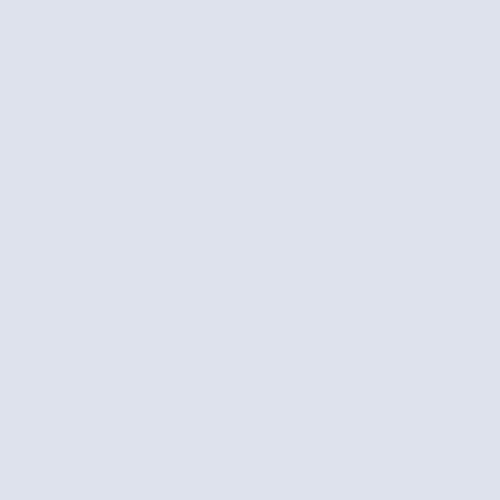A blank, grey square box is depicted. All four sides of the box, top, bottom, left, and right, are equal in length, forming a perfect square. The uniformity of the box's dimensions emphasizes its symmetry and simplicity.